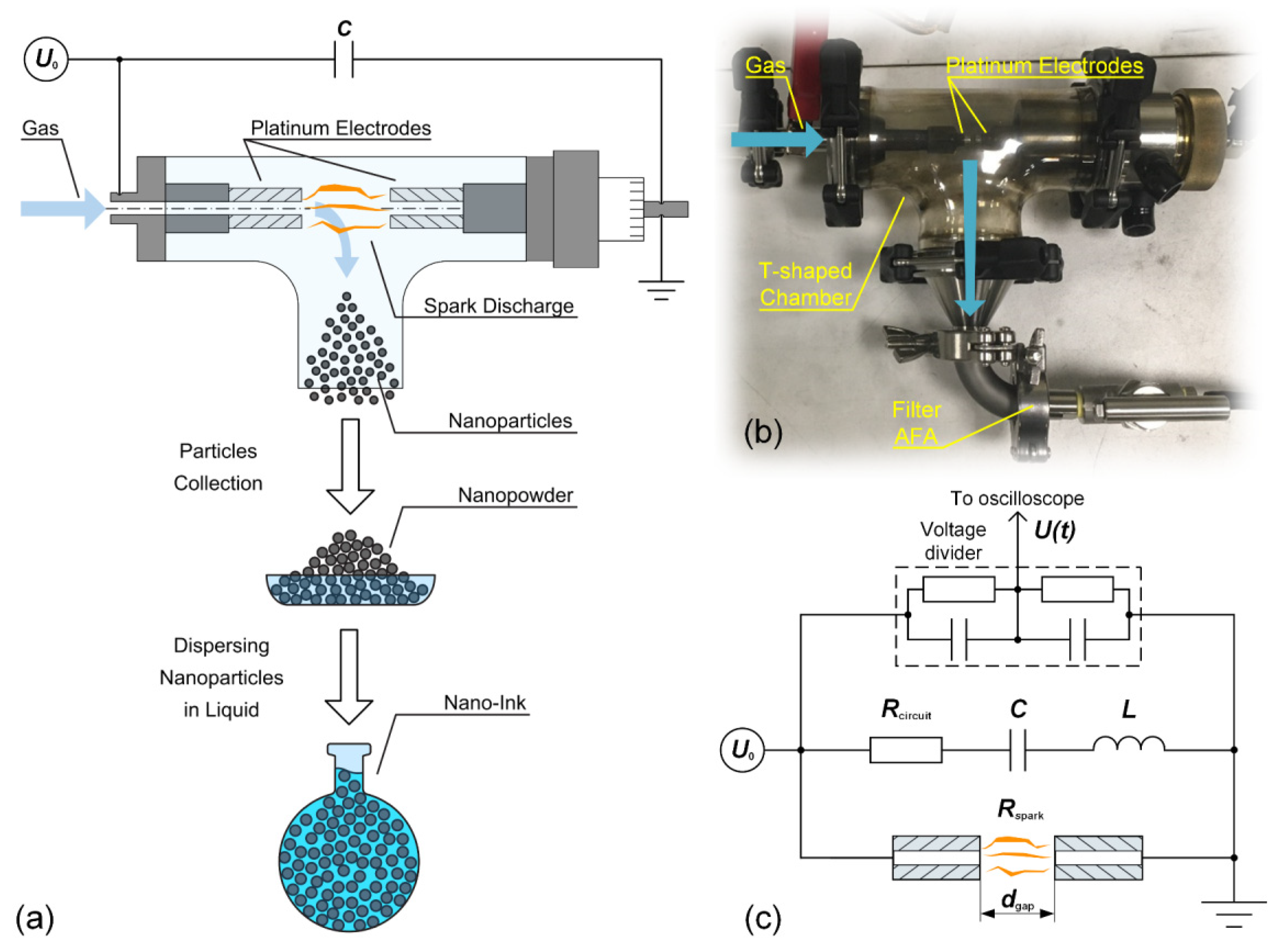The image is a detailed instructional diagram explaining the functionality of a specialized device used for generating and collecting nanoparticles, possibly for creating nano ink. On the left half of the image (Figure A), a detailed line drawing illustrates the internal workings of the device. It shows a platinum electrode spark discharge mechanism, where nanoparticles are generated and subsequently collected in a small dish, labeled "particles collection." These nanoparticles are then dispersed into a liquid to form nano ink.

The top right part of the image (Figure B) features a real-life photograph of the device, resembling a pipe setup. This figure is labeled with terms such as "gas," "platinum electrodes," "T-shaped chamber," and "filter AFA," all highlighted in yellow font. Blue arrows indicate the flow direction within the device. Figure C, situated in the lower right segment of the image, contains additional diagrams and instructions detailing an "oscilloscope voltage divider" setup, showcasing how voltage and sparks are managed within the system, emphasizing the charge distribution and circuit functions.

Together, these elements provide a comprehensive understanding of how the device operates: from gas intake and spark generation to nanoparticle collection and the eventual formation of nano ink.